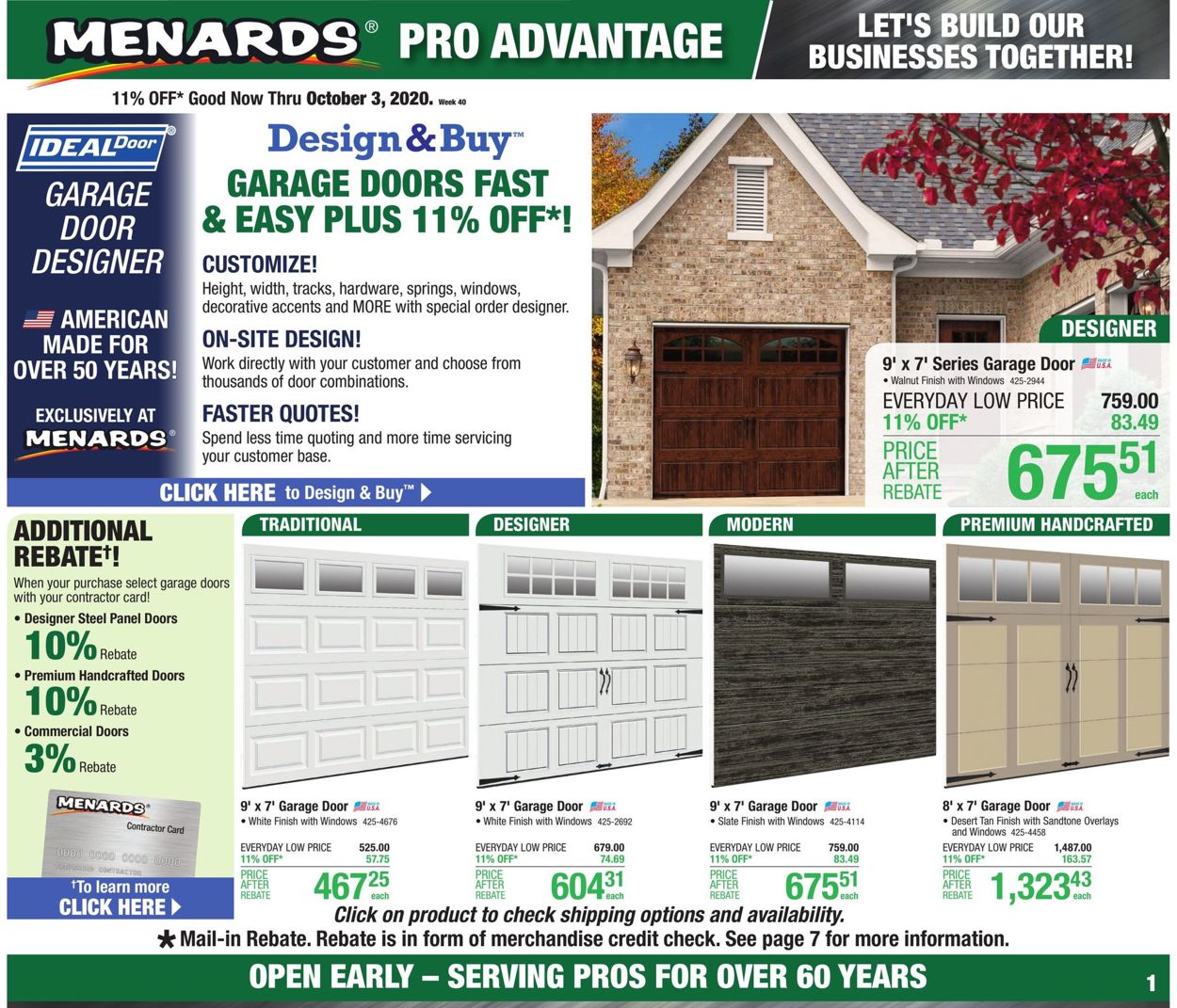This detailed caption describes a screenshot of an advertisement layout. 

---

The horizontal screenshot captures an advertisement for Menards, featuring structured banners and various elements on a clean, white background. The top part of the ad has a green and gray banner, while the bottom section prominently displays a green banner. In the upper left corner, the Menards logo is shown in bubble text set against a rainbow-colored background, with the tagline "Menards Pro Advantage: Let's build our business together" positioned adjacent to it.

Prominently displayed on the lower portion of the ad are images of four different types of garage doors: Traditional, Designer, Modern, and Premium Handcrafted. Each type is labeled accordingly, providing a clear distinction between them. 

Towards the top right corner of the image, there is an additional photograph depicting a brown garage attached to a stone house with a gray roof. This particular 9-foot by 7-foot garage door is priced at $675.51.

Adjacent to this, on the left side, a vertical column highlights the "Additional Rebate" section, outlining the rebates offered. 

A Menards Contractor Card is also displayed, accompanied by a button inviting viewers to "Learn More, Click Here." Pricing details for various garage doors are scatter throughout; for example, some prices include $467.25, $604.31, and $675.51, with the Premium Handcrafted garage door listed at $1,323.43.

Lastly, the bottom green banner asserts Menards' dedication with bold white text: "Open early, serving pros for over 60 years."

---